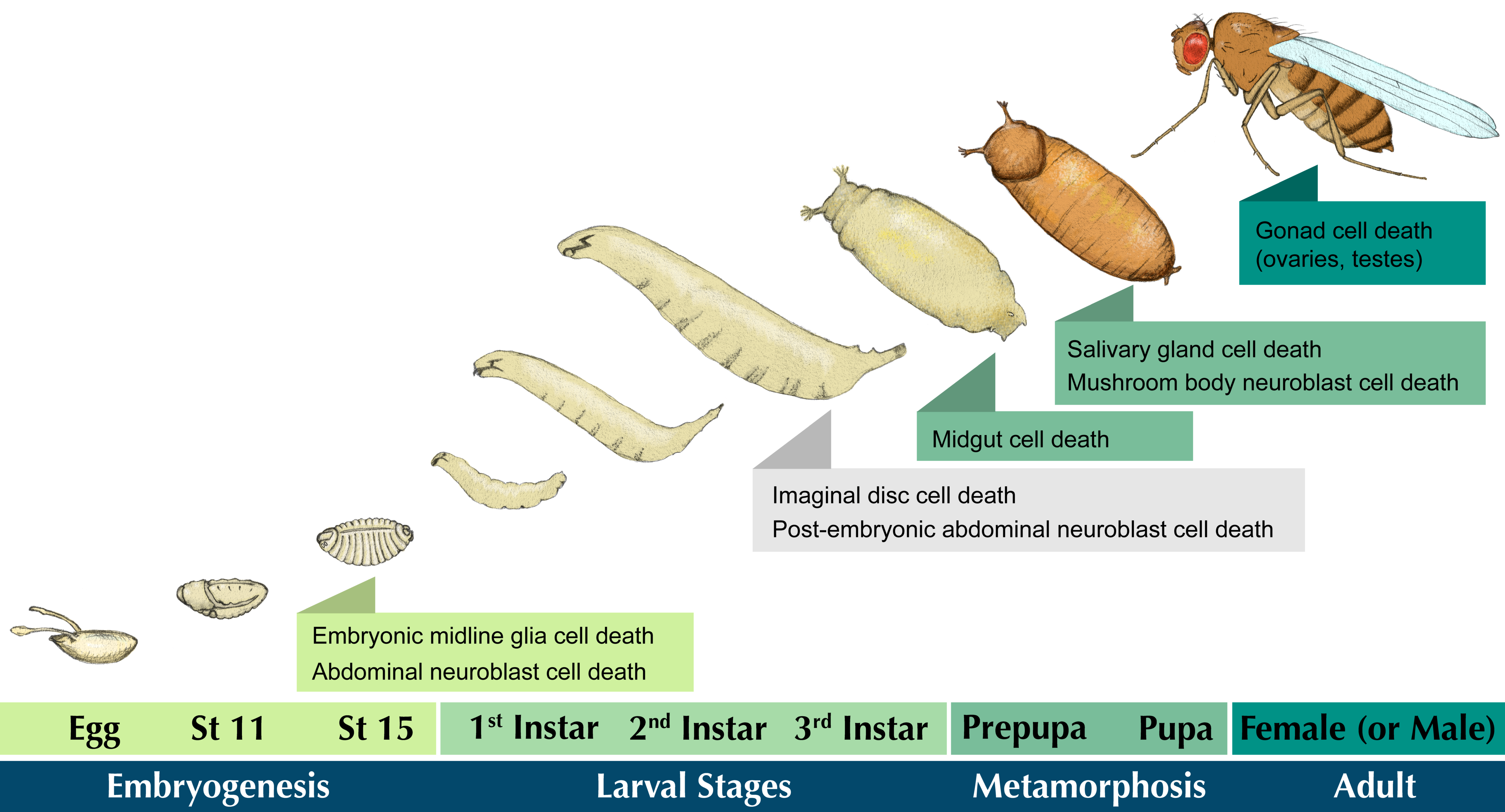This detailed chart, likely suited for a biology class, meticulously illustrates the developmental stages of an insect, possibly a fly, from egg to adult in nine distinct phases. The horizontal axis features a blue band categorizing the stages into embryogenesis, larval stages, metamorphosis, and adulthood. The embryogenesis stage is broken down further into sub-stages: egg, S411, and ST15. Following this, the larval stages are depicted with first, second, and third instar phases, all showcased in varying shades of green. As development proceeds, darker green sections represent the prepupal and pupal stages, culminating in the final adult stage differentiated by male or female in the darkest green. 

Each stage is accompanied by detailed illustrations, beginning with the smallest egg and evolving through the larval stages — depicted with three white forms featuring black lines — into more defined insect forms that change from yellow to orange, and finally into a fully mature insect, resembling a wasp. Additionally, the chart provides intricate information regarding cell death processes at each stage: the embryonic midline, gonad cells (ovaries and testes), salivary glands, mushroom body neuroblasts, mid-gut, and imaginal discs, all color-coded and organized in a clear vertical progression. This comprehensive visualization effectively captures the developmental transformations of the insect lifecycle, making it an invaluable educational tool.